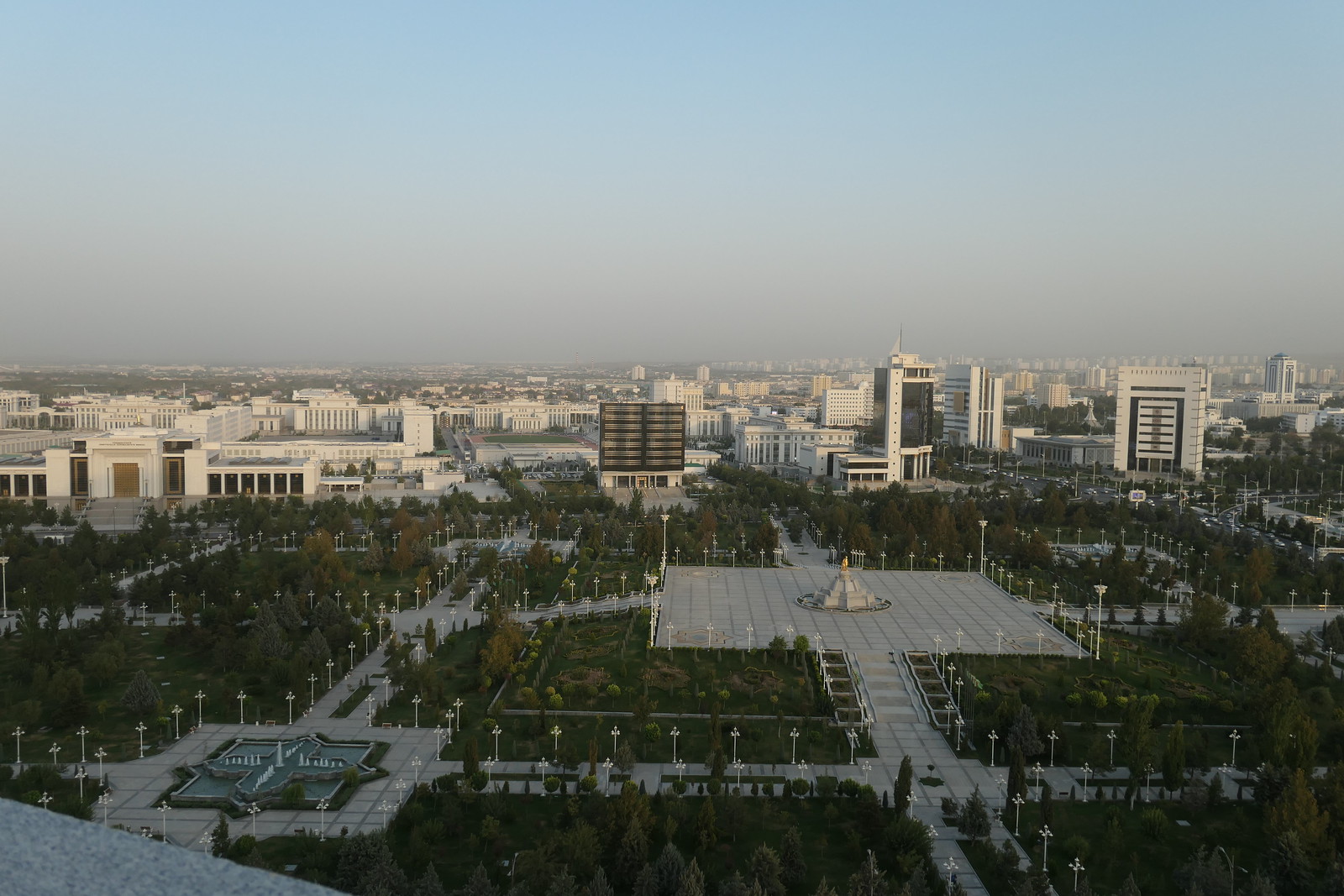The photograph is a high-altitude, wide-angle view of a sprawling city, possibly taken from a tall building or a drone. The foreground features a meticulously landscaped park laid out in a grid-like design with numerous shrubs, lined trees, and hundreds of white light poles. At the center of this park is a large concrete square featuring a star-shaped fountain, around which stands a gray monument crowned with a golden statue. In the background, the cityscape extends to the horizon, filled with a variety of buildings, including many high-rises. The sky above is a dusty blue, slightly obscured by a layer of pollution or fog. The buildings further in the distance have a stark white or cream appearance, contributing to the sense of depth and vastness in the photo.